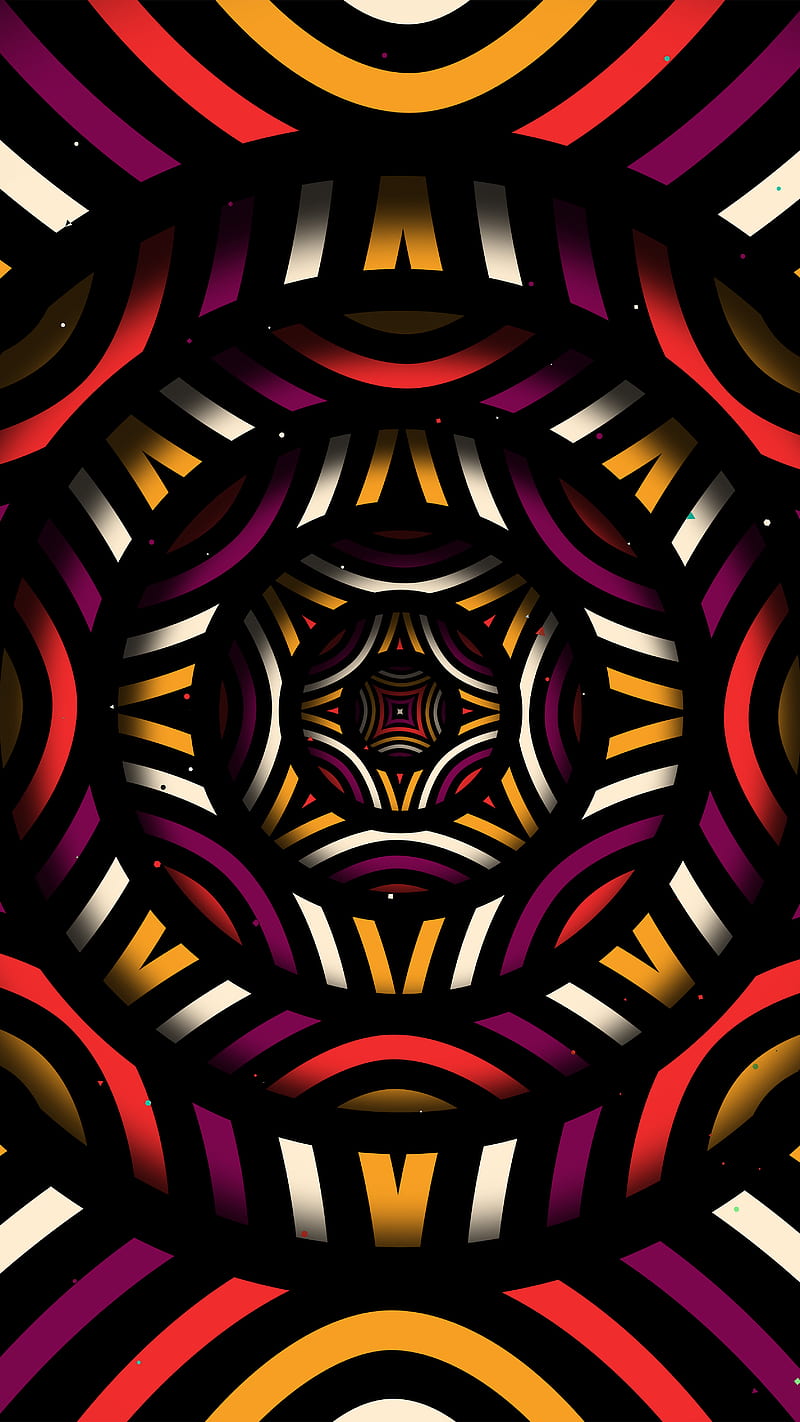This image is a captivating and detailed digital design in portrait orientation, featuring a mesmerizing pattern that resembles a kaleidoscope or sacred geometry. It is composed of numerous concentric circles, each bordered with black and filled with vivid colors such as purple, red, orange, yellow, and white. These circles start large in the center and progressively decrease in size as they radiate outward, creating a sense of expansion and a subtle 3D effect. The pattern within each circle is intricate, with curved lines and rings that shift and change colors rapidly, adding to the psychedelic and dynamic feel of the design. This visually striking piece ultimately forms a star-like shape, embodying a complex and ever-changing tapestry of colors and forms.